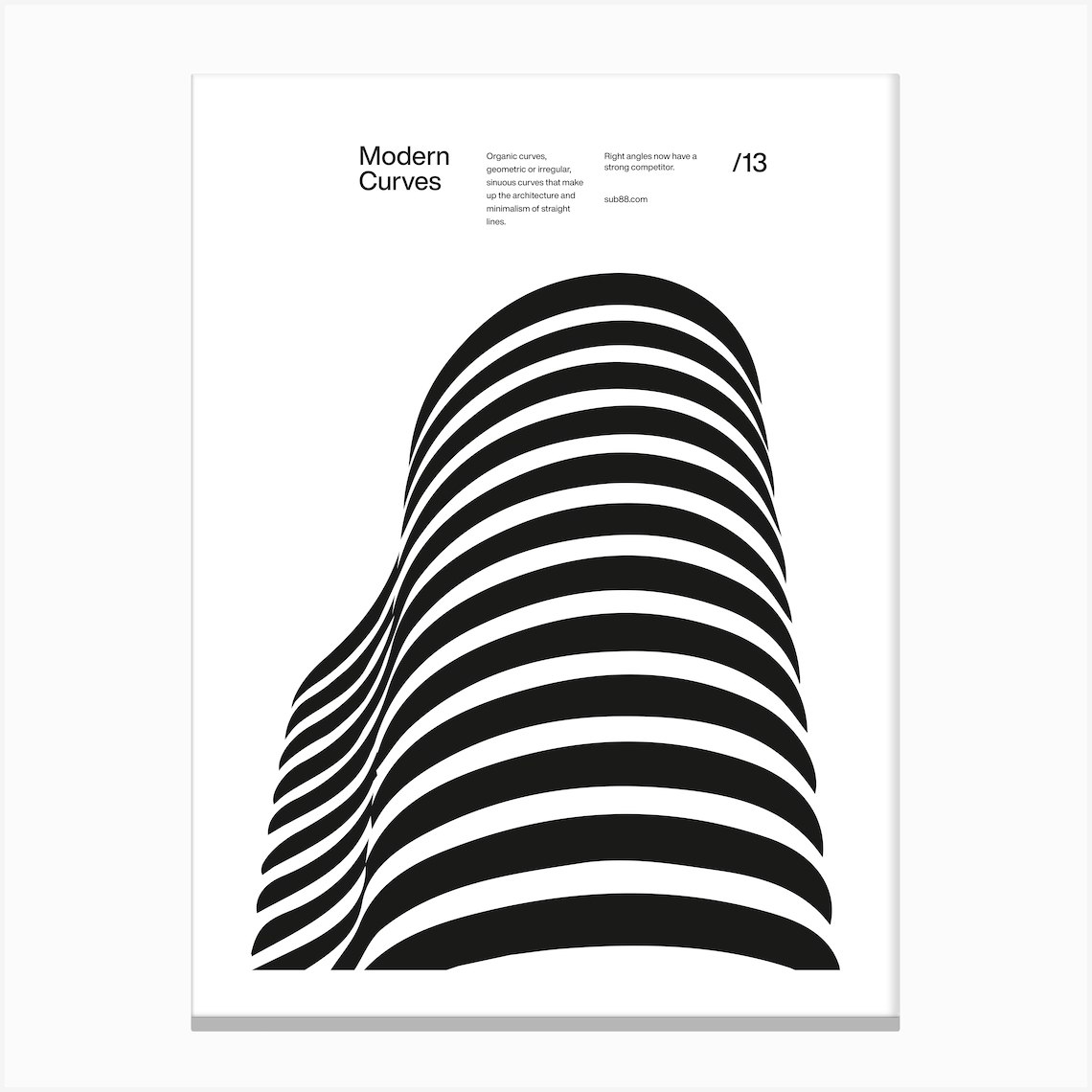The image features a stylistic and abstract rendition of a building, dominated by black and white stripes curving upward in a wavy motion, evocative of a zebra pattern. At the very top, the words "Modern Curves" are prominently displayed on a white background. To the right of this title, in a smaller font, the following text appears: "Organic curves, geometric or irregular, sinuous curves that make up the architecture and minimalism of straight lines. Right angles now have a strong competitor." There's also a URL listed as "sub88.com" and the number "13" following a forward slash. The image consists of twelve distinct black stripes, interspersed with white, beginning and ending with black, creating a dynamic sense of movement and contrast throughout the composition.